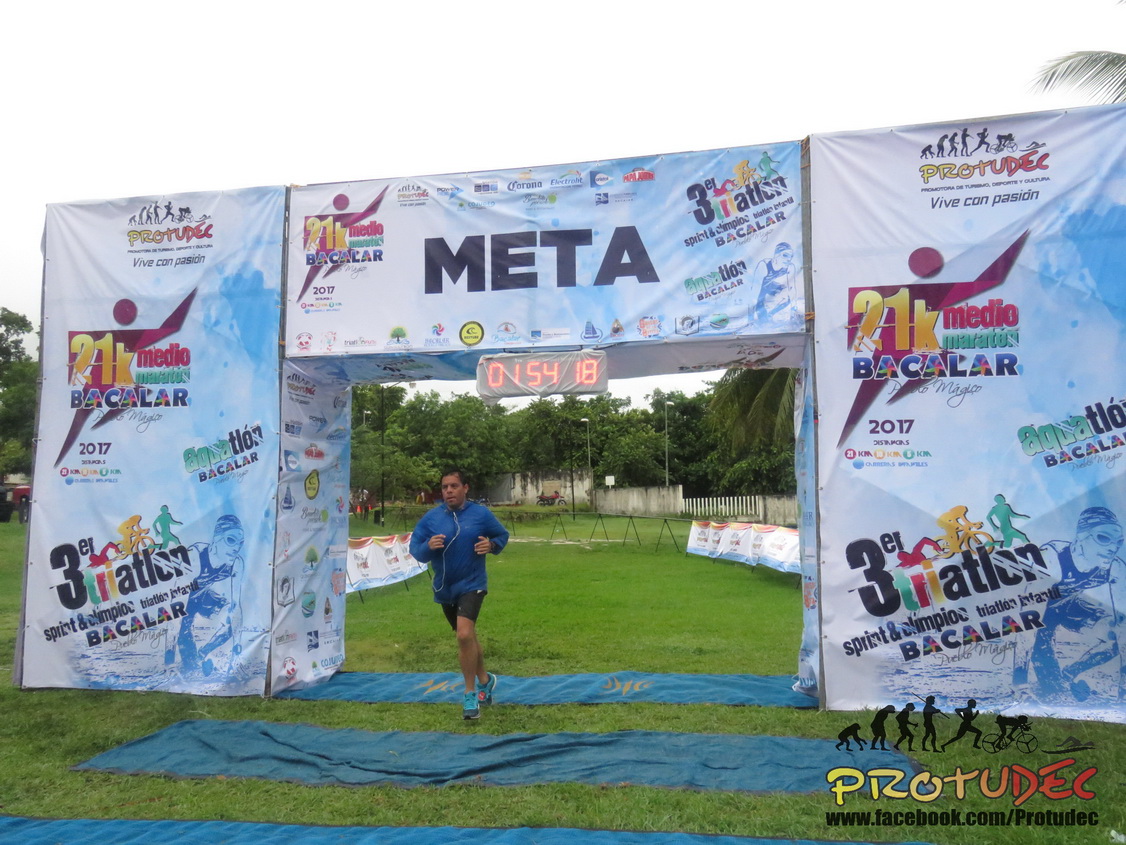This photograph captures a man completing a race by running past the finish line. The finish line is marked by a rectangular passageway created by three columns: two vertical ones on the left and right, covered in fabric graphics of a running person, and the text "21KBACALAR" and "3TRIATHLONBACALAR" at the bottom corners. These vertical columns are connected by a horizontal section at the top, which is marked with the text "META" and houses a digital clock displaying "01:54:18." The man is dressed in a blue jacket, black shorts, and blue shoes, running over blue mats presumably placed for safety. In the lower right corner of the image is the text "PROTUDEC" alongside a graphic of a running man. The backdrop features a grassy field and trees, under an overcast sky. The overall scene captures the triumphant moment of crossing the finish line, set against a vibrant outdoor environment.